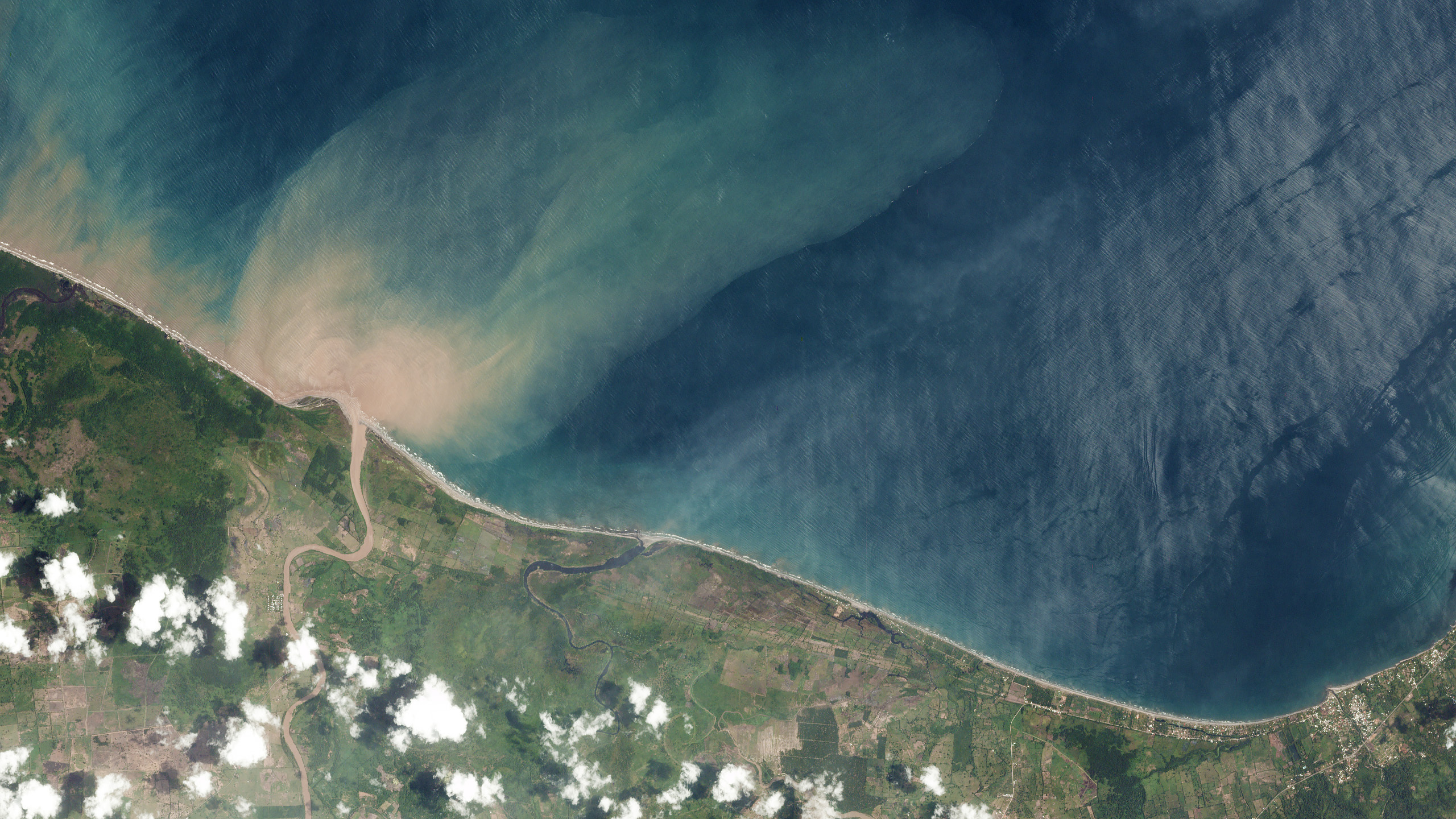An aerial view photograph showcases a striking landscape where two-thirds of the image is dominated by a calm body of water, likely an ocean or a large lake, featuring a spectrum of blues from deep royal to aqua with light cream swirls. The water appears still and tranquil, meeting the land with a distinct, white, stringy coastline resembling a beach. The lower third of the photo captures varied land, a mix of lush green and earthy browns, traversed by a winding, wavy dirt road extending from the shoreline toward the bottom of the frame. Dotted across the land are numerous bright white clouds in various shapes and sizes, giving the impression of both clouds and possibly flowering trees. The photograph, possibly taken from an airplane, also shows minute details suggestive of small buildings in the lower right corner, further emphasizing the aerial perspective.